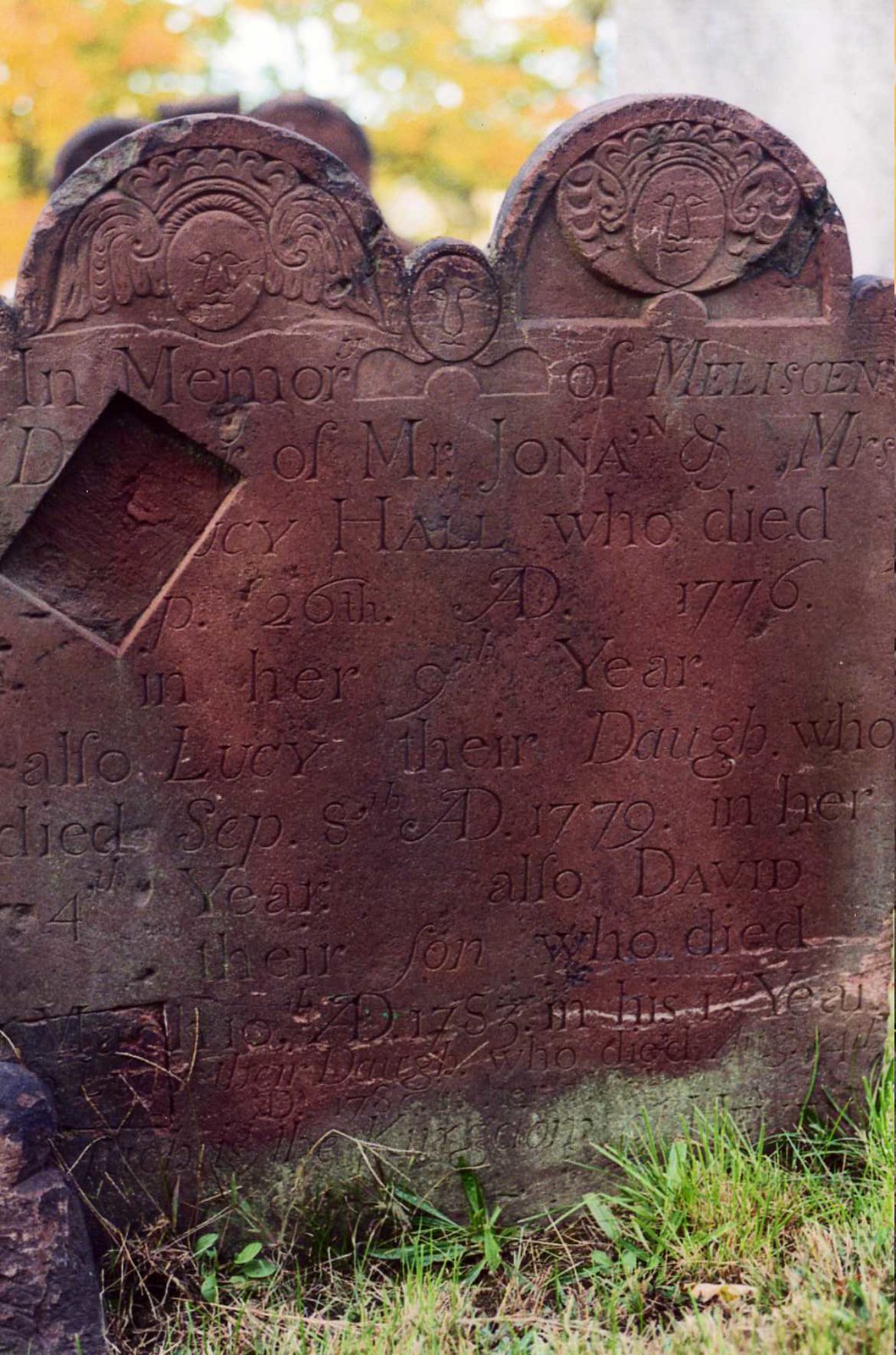The image depicts an outdoor scene featuring an old, weathered tombstone, distinct in its reddish, beet-red hue with a greenish-grey base. The sky above is gray and slightly blurry, and the background is filled with blurry fall foliage in shades of yellow and green. The tombstone itself is unique, made of a reddish material reminiscent of red clay, with two curved protrusions at the top, each adorned with carved images—one of an angel and the other possibly of a royal figure. Part of the tombstone appears to have a chunk missing, shaped somewhat like a wallet or soap bar, which cuts out some of the engraved words. Despite the damage, the inscription reads "In memory of ..." with a fragment of the name "Melliscens," though the entirety is not legible. Names like Mr. Jonah, Mrs., and Lucy are partly visible, with dates from the 1700s, including 1776 and 1779. The grass and natural light add to the serene, autumnal ambiance, enhancing the historical and melancholic atmosphere of the scene.